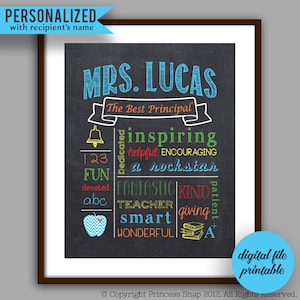The advertisement features a computer-generated image showcasing a personalized framed plaque with a darker gray background. The frame, which has a black outline and a white border, prominently displays “Mrs. Lucas” in blue chalk-like letters centered in a black rectangle. Below this, there's a blue banner proclaiming "The Best Principal." Surrounding the central text are an array of colorful, inspiring words: "inspiring" in green, "encouraging" in yellow, "a rock star" and "smart" in blue, "wonderful" in orange, "dedicated," "helpful," "fantastic," "teacher," "kind," "giving," and "patient." 

Additional educational motifs enhance the design: a yellow bell with numbers "123," the word "fun," "ABC," and a bluish apple adorn the frame, emphasizing the teaching theme. The top left corner of the frame features a banner that reads "Personalized with recipient’s name," while a blue circle at the bottom right corner states, "Digital file printable." Lastly, a small credit at the bottom denotes "Copyright Princess Snap 2012."